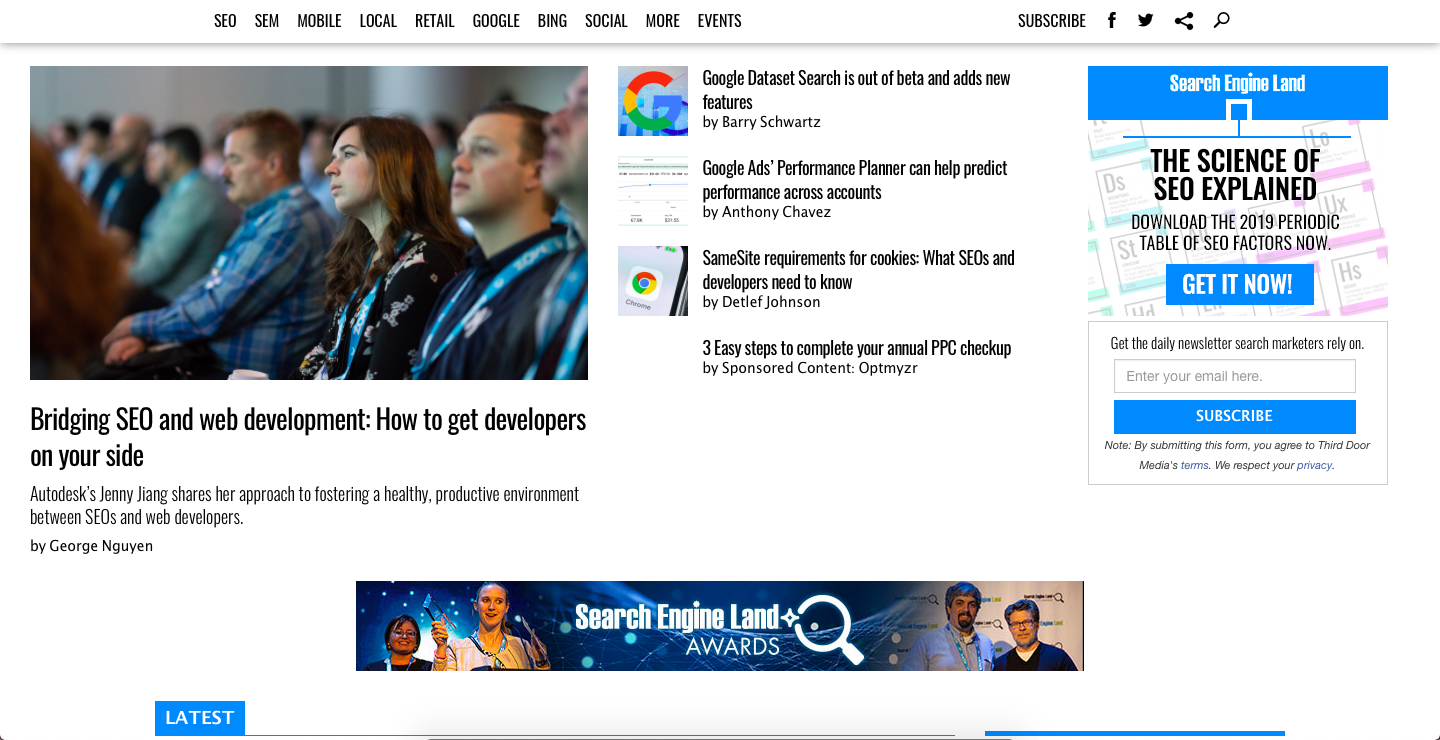The image illustrates a webpage with a clean, white background featuring a combination of text, images, and logos. At the top section of the page, a menu bar displays keywords such as "SEO," "SEM," "mobile," "local," "retail," "Google," "Bing,” "social," "more events," and "subscribe." On the right side of this menu, notable elements include the Facebook and Twitter logos, a Settings button, and a magnifying glass icon indicating a search function.

On the left side of the page, there's a prominent image depicting approximately 40 to 50 people seated in what appears to be a conference room. These individuals seem to be engaged in a presentation or listening to a speaker.

Beneath this image, a headline reads: "Bridging SEO and Web Development: How to Get Developers on Your Side," authored by George Nguyen with insights from Autodesk's Jenny Jing about promoting a cooperative and productive relationship between SEOs and web developers.

On the right side of the page, a list of article titles is displayed, including:
- "Google Dataset searches out of beta and adds new features” by Barry Schwartz.
- "Google Ads Performance Planner can help direct performance across accounts” by Anthony Chavez.
- "Same-site requirements for cookies: what SEOs and developers need to know” by Detlef Johnson.
- "Three easy steps to complete your annual PPC checkup" by Sponsor Content Optimizer.

Additionally, there is an advertisement for Search Engine Land titled "The Science of SEO Explained," featuring a call-to-action button labeled "Get Now" to download the 2009 periodic table of SEO factors. Below this, another banner promotes the Search Engine Land Awards.

At the bottom left corner of the page, there's a section labeled "Latest." Overall, the design is minimalistic, featuring black text on a white background with relevant images accompanying each article and advertisement.